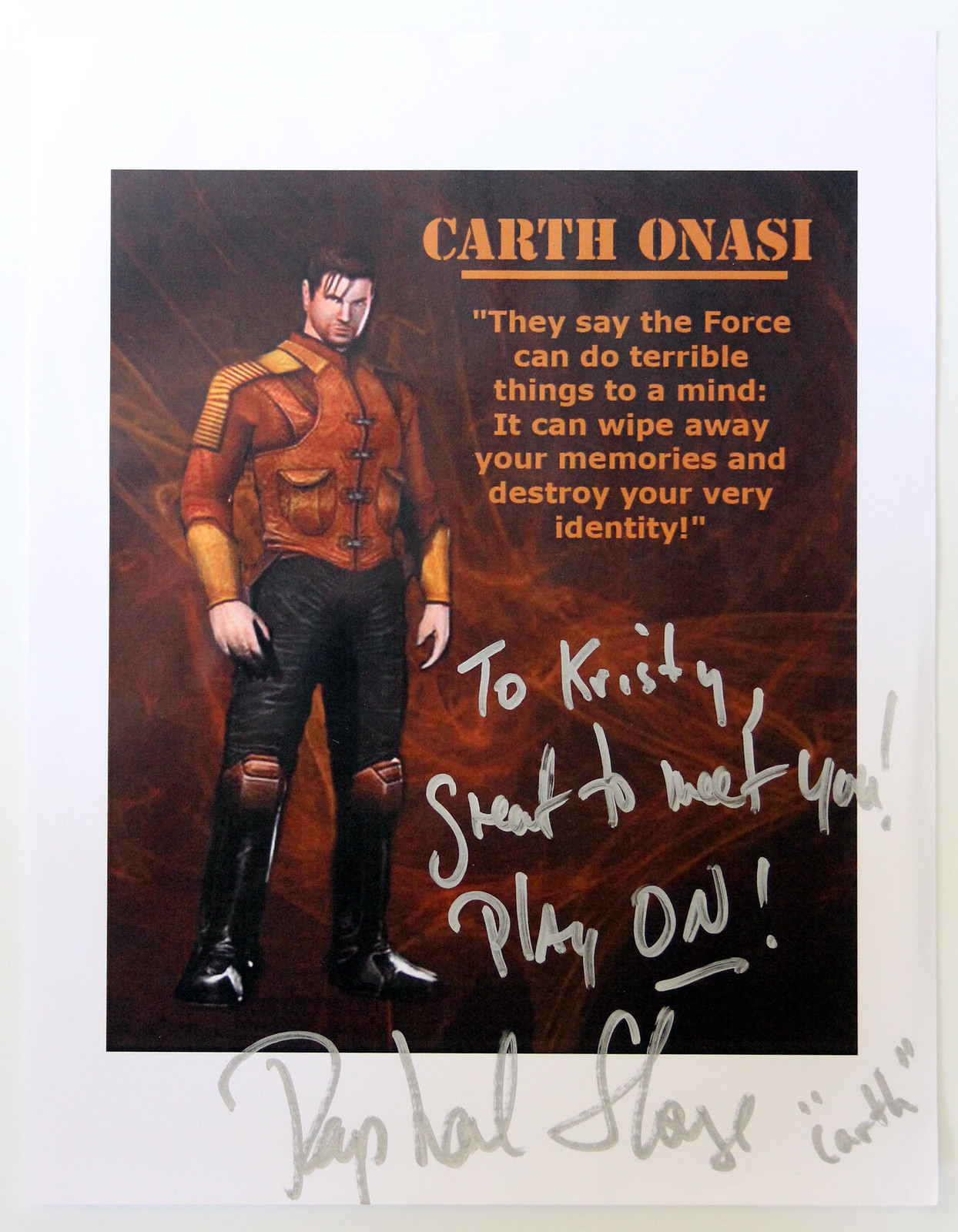The image features a poster with a brownish-orange background depicting dark flame-like graphics. The centerpiece is an illustrated character, possibly from a video game or comic, named Karth Onasi. He is portrayed with brown hair, wearing a leather vest, black pants, brown knee pads, yellow armbands, and likely boots. His hands are visible, emphasizing his dynamic pose. To the right of the character, the text at the top reads "Karth Onasi." Below that, a quote states: "They say the Force can do terrible things to a mind. It can wipe away your memories and destroy your very identity." Beneath the quote, a handwritten inscription says, "To Christy, great to meet you. Play on," followed by a signature, possibly reading "Raphael Stage Garth" and including a brief additional note, "Karth."